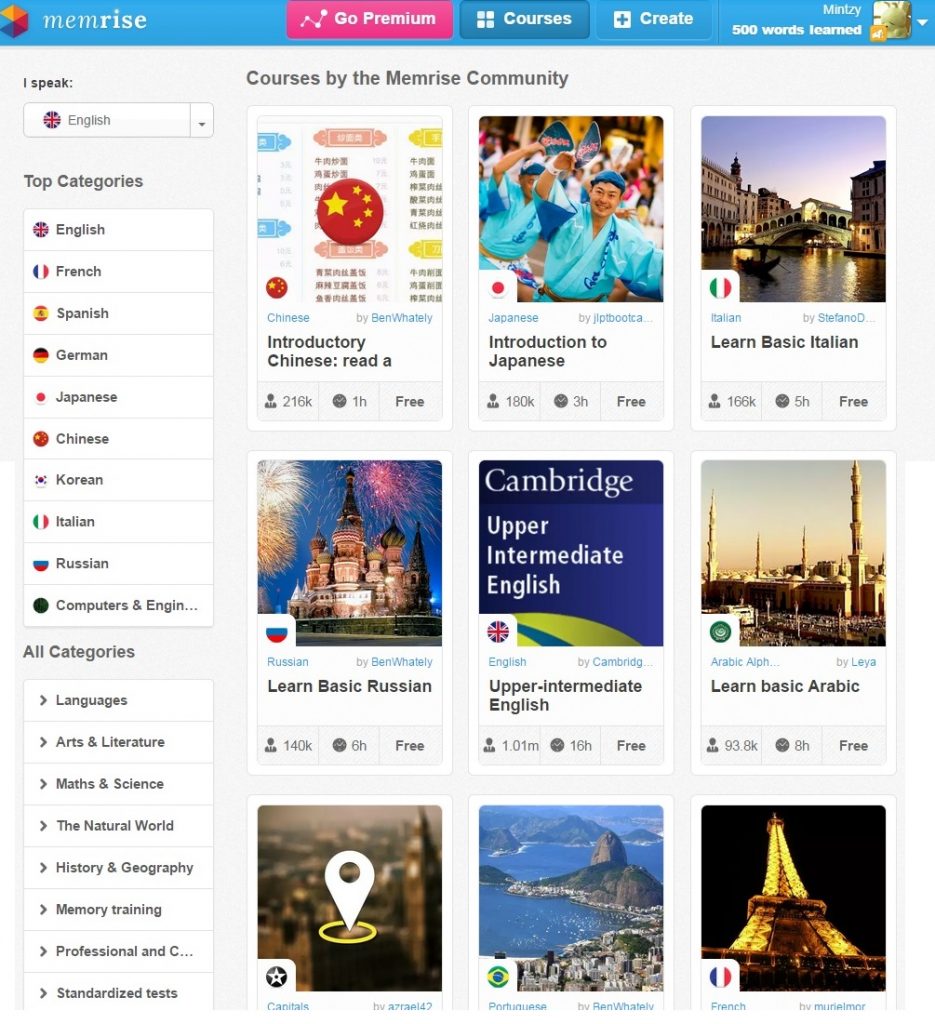This is a cropped screenshot of the Memrise website's interface. The header features a thin blue bar at the top. On the right side, there is a pink box labeled "Go Premium." Next to it, in a darker blue box, is the word "Courses." Further right, small white font spells out "Create." Continuing to the right, the user profile is displayed, showing that 500 words have been learned in small white font beneath the user's icon.

The main body of the page is predominantly gray on the left. At the top left, small black letters spell out "I speak," accompanied by a drop-down box currently set to English. Below this, the section title "Top Categories" is presented in bold gray font. Vertically listed beneath it are various languages: English, French, Spanish, German, Japanese, Chinese, Korean, Italian, Russian, followed by the category "Computers & Engineering."

Further down, "All Categories" is displayed in dark gray font with another vertical list of categories, each marked with an arrow on the left to expand the category. On the right side of the page, the heading "Courses by the Memrise Community" appears. Below this, the interface showcases thumbnails of different courses. The layout features three courses per row, with nine courses fully visible on the screen.